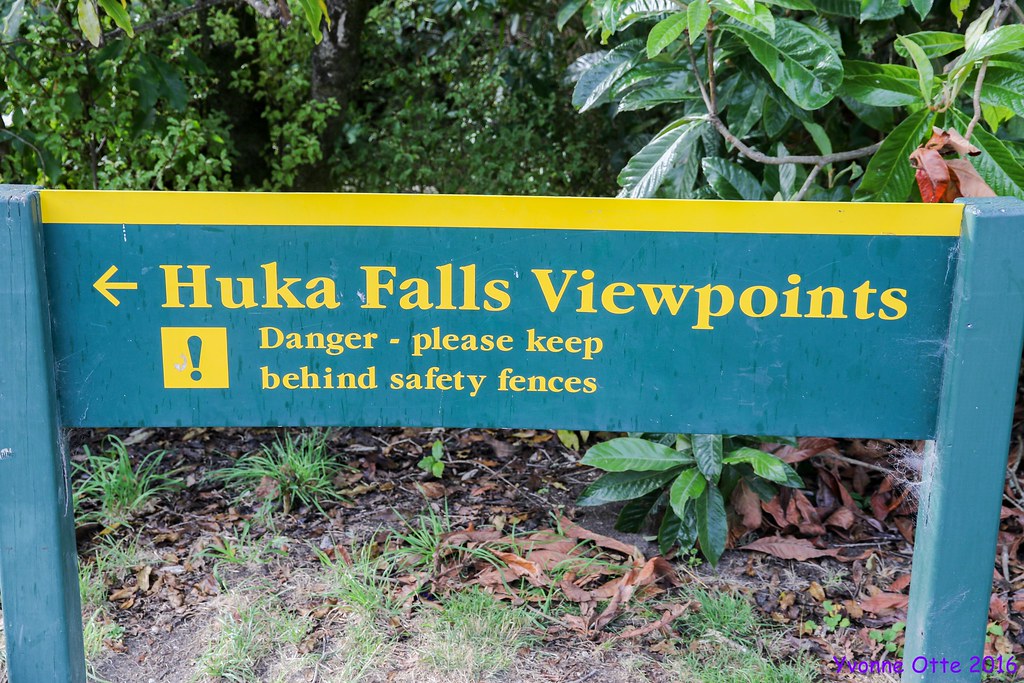In this image, a cautionary sign stands prominently in front of a scenic outdoor area. The sign is supported by two teal wooden posts and features a teal rectangular panel with a yellow border at the top. Large yellow text on the sign reads "Huka Falls Viewpoints," while smaller text beneath it warns, "Danger! Please Keep Behind Safety Fences!" accompanied by a yellow exclamation mark within a square on the left side of the text. Cobwebs can be seen clinging to the sides of the sign, adding a sense of age and weathering. The scene is surrounded by lush, tropical vegetation including large green shrubs and palm leaves, and the ground below is strewn with gray dirt, fallen leaves, and new grass shoots. In the bottom right corner of the image, the name "Yvonne Ott 2016" is credited in purple, likely indicating the photographer. The setting appears to be taken during daylight hours.